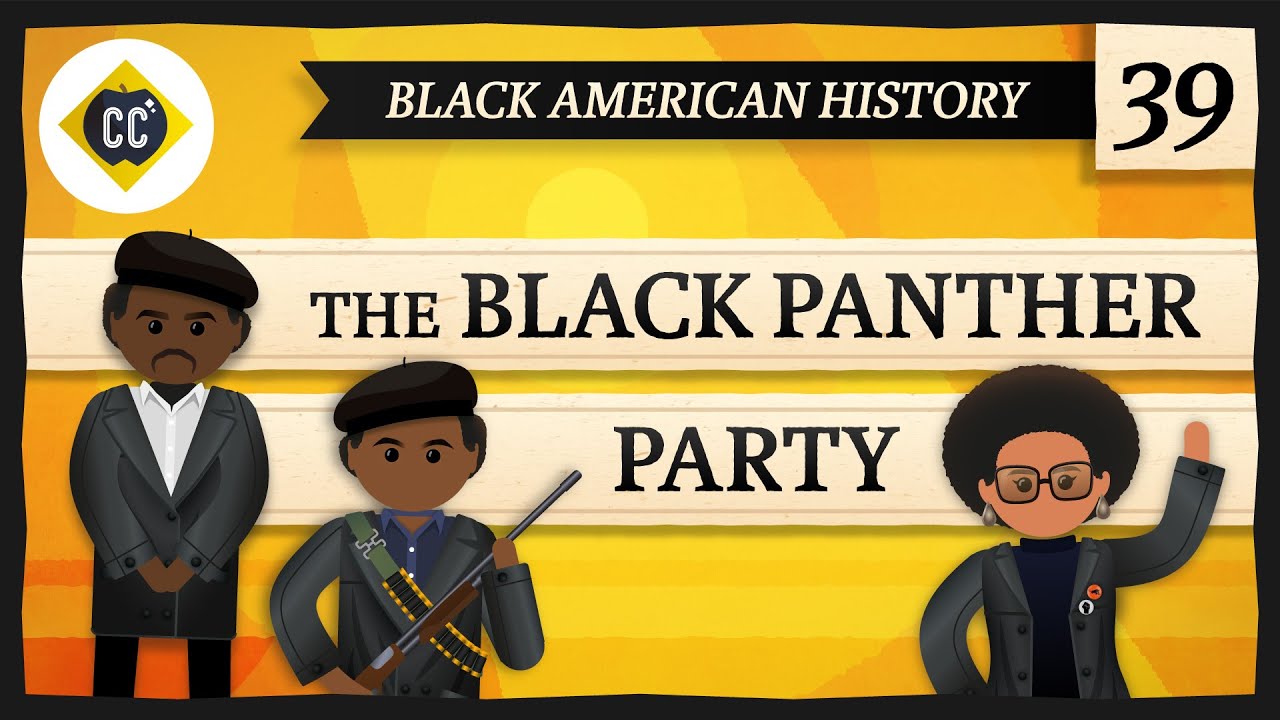This is a digital illustration, possibly a Crash Course thumbnail for Episode 39 of Black American History, featuring the Black Panther Party. The scene is set against an orange and white patterned background surrounded by a black frame. In the top left, there's a white circle with a yellow diamond inset, overlaid by a black apple with white text reading “CC”. The top right contains a tan square with the black number "39". 

To the left, a horizontal black stripe resembling a bookmark features the tan text "Black American History". Below this, two black horizontal strips serve as banners; the top one reads "The Black Panther" and the one beneath it says "Party". 

Three figures stand in front of these banners: 
- On the left is a man with dark brown skin wearing a black beret, black jacket, and white shirt.
- To his right is another man with slightly lighter skin, also in a black beret and similar jacket, with a blue shirt. He has a green ammunition strap across his chest and is holding a shotgun.
- On the far right is a woman with a large afro, dark skin, black square glasses, and teardrop-shaped earrings. She’s dressed in a black jacket adorned with a white and orange button and possibly other pins.

The entire composition conveys significant elements of the Black Panther Party and highlights key figures of the movement.